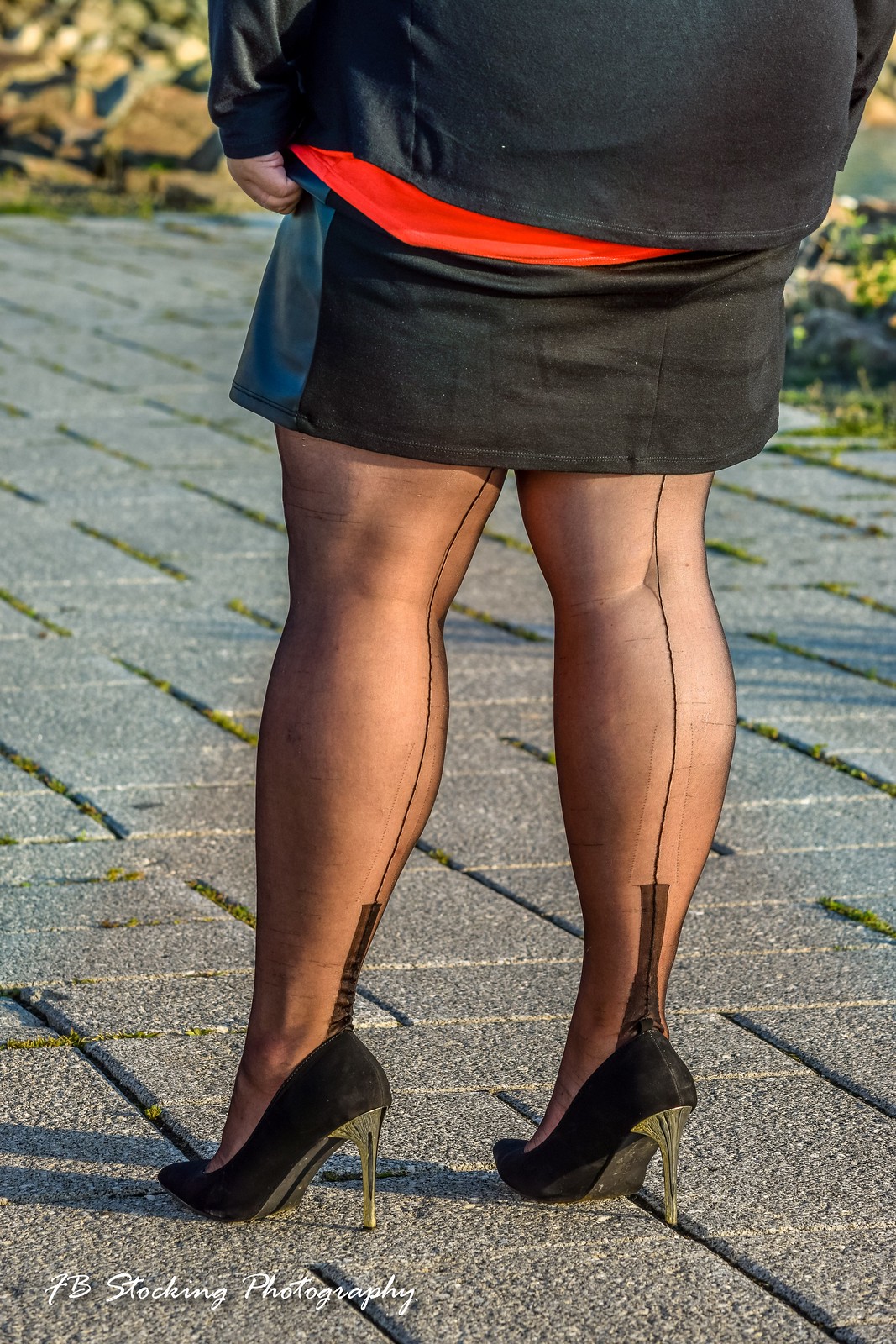The image shows the legs of a medium-built Caucasian woman standing outside on concrete tiles. She is wearing a black skirt, black high-heeled shoes with a silver heel, and sheer black stockings with a distinct thin line running up the back. The photo captures her from just above the knees downward, focusing on the back of her legs and her high heels. The setting is outdoors, and there is text in the lower left corner reading "FB Stalking Photography."